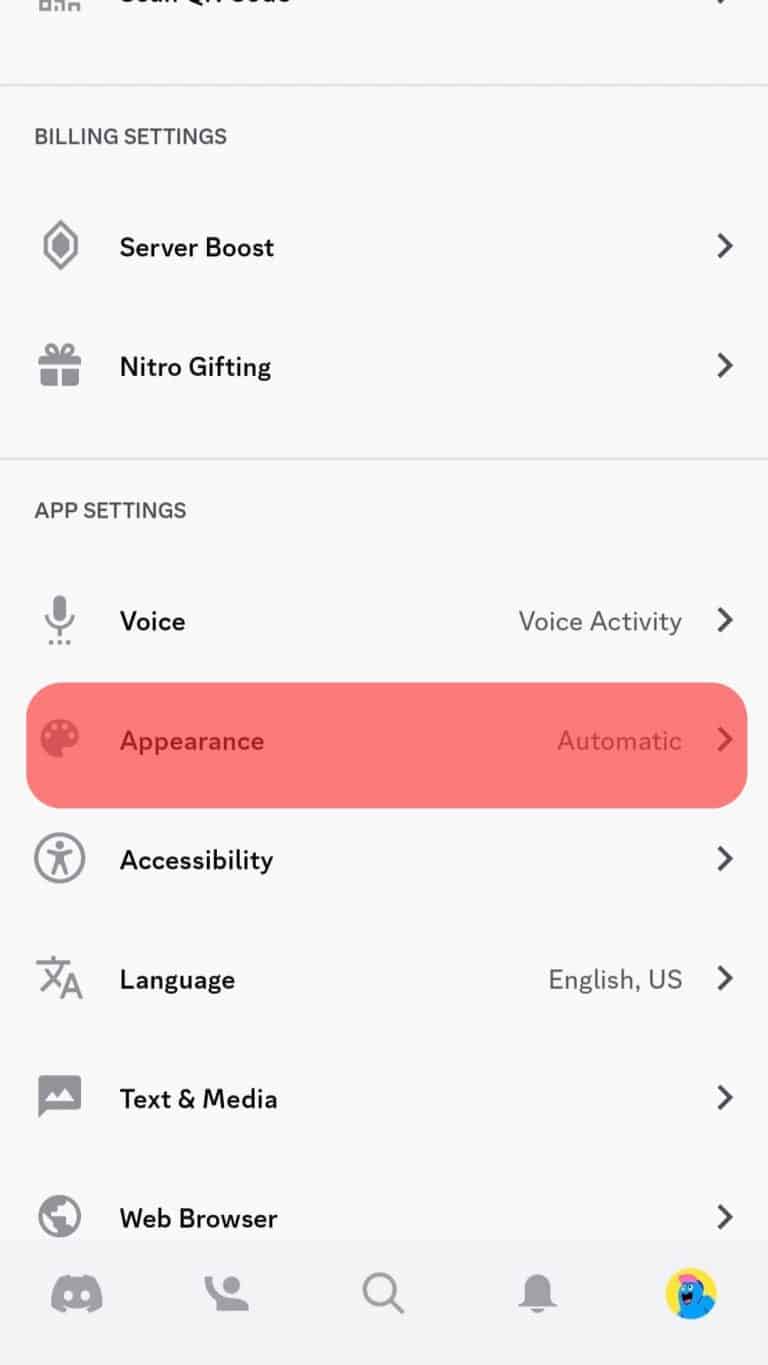The image depicts a smartphone screen in portrait orientation showcasing a user interface, presumably from a mobile application. At the very top, there is a partially cut-off section followed by a gray line beneath it. In uppercase gray text, it reads "BILL SETTINGS." Right below, within a diamond-shaped icon, the words "Server Boost" are displayed, with a gray arrow pointing to the right. Next, the text "Nitro Gifting" is accompanied by a small gift icon, also in gray. 

A horizontal divider line separates this section from the next, which is titled "APP SETTINGS." In black text, the word "Voice" appears alongside a gray microphone icon. To the right, it reads "Voice Activity." Further down, the text "Appearance Automatic" is observed within a reddish, rounded rectangle featuring an artist palette icon. 

Continuing down, the section titled "Accessibility" includes an icon of a person inside a circle. Following that, the "Language" section displays an 'A' character and a kanji character to the left, with "English (US)" written to the right. Lastly, the text "Text and Media" is presented next to a small landscape icon, followed by "Web Browser" paired with a globe icon.

At the bottom left of the screen, various icons are visible: the Discord logo, a person, a magnifying glass, a bell, and an image of a character with a blue background.